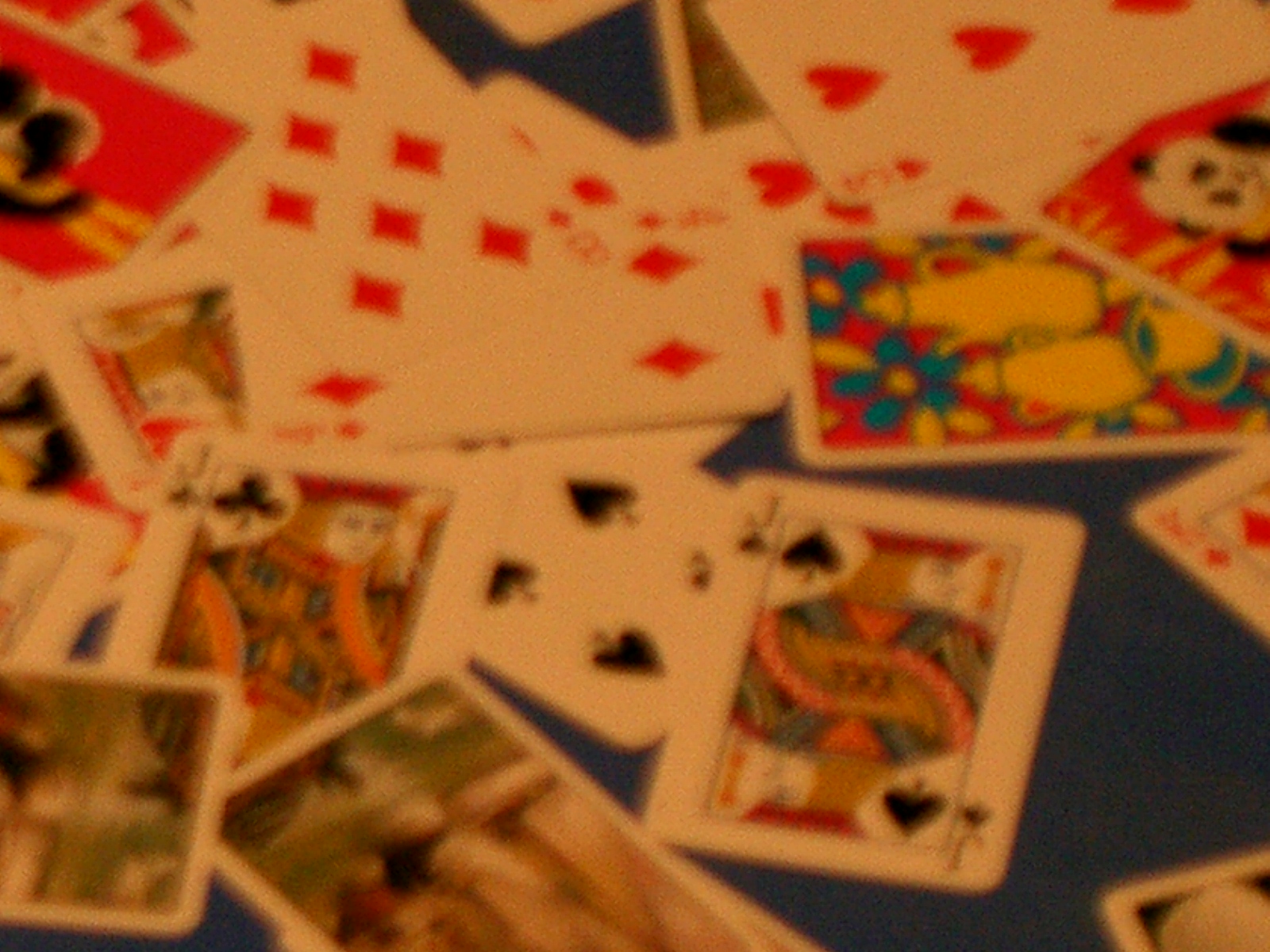In this image, playing cards are scattered across a blue surface that resembles a dealer's station at a Las Vegas blackjack table. Among the array of cards, the jack of hearts, the four of spades, the jack of clubs, a joker, the three of hearts, and the king of spades are all distinctly visible. The cards are in varying orientations, with some face up and others face down. There are multiple jacks in the image, with the jack of hearts and jack of clubs both being black in color, while the king of spades is red. Notably, the backside of some cards, possibly depicting a panda bear, suggests a unique card design. Additionally, two jokers are visible at the bottom of the image, further adding to the assortments of cards. The scene presents a chaotic yet intriguing display reminiscent of a lively card game.